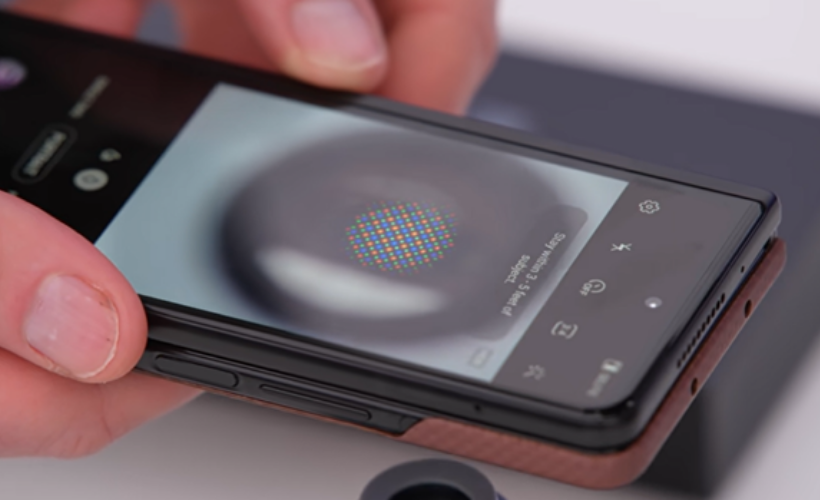A professionally taken close-up photograph captures a white man's hands, with visible pink skin and unpainted, jagged fingernails, holding a smartphone that appears to be either an Android or Samsung device. The smartphone, encased in both a black inner case and a light brown outer wallet case, features a screen displaying a gray orb surrounded by white text, which is difficult to discern. The phone screen exhibits a pattern with alternating polka dots in blue and orange. The hands firmly grip the phone with one positioned on the upper left and the other on the lower left side, and there are visible black buttons. The background is a blurred mix of white and gray, casting a shadow of the phone and hands.